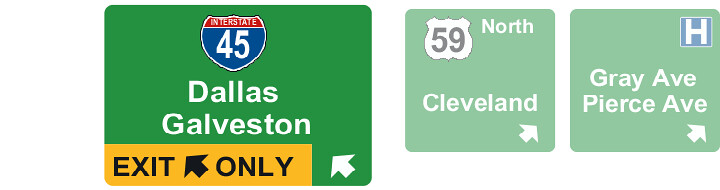Set against a white background, the image showcases three photoshopped street signs. 

- On the left, there is a rectangular green street sign. At the bottom left corner of this sign, against a yellow backdrop, "EXIT ONLY" is displayed in black print, accompanied by an upward diagonal arrow. Above this, the sign reads "Dallas-Galveston" in white print. Prominently positioned at the top center, "Interstate 45" is presented in red, white, and blue.

- In the middle, a pale green square sign reads "59" signifying the road number for a northbound route. Below this, "Cleveland" is written, with an arrow in the lower right corner pointing diagonally upwards to the east.

- On the right, a green square sign displays "Gray Ave Pierce Ave" with an arrow pointing diagonally upward to the east. Additionally, in the right-hand corner of this sign, there is a dark blue letter "H," indicating a hospital.